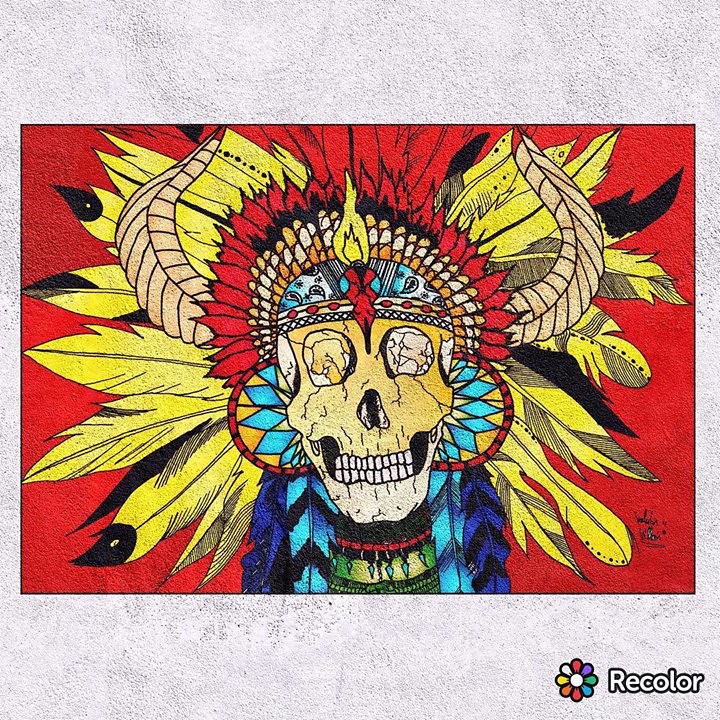This image features an intricately detailed, vibrantly colored drawing of a skull adorned with a headdress reminiscent of a Native American Indian chief's attire. The skull itself is depicted in light yellow hues and is framed by a pair of ram-like horns that curve outward and then inward. The headdress is an elaborate display of multicolored feathers, including shades of yellow, red, turquoise, blue, purple, and some with black tips, arranged symmetrically. The skull also sports large circular hoop earrings in red, blue, and beige, with long feathers in dark blue and light blue hanging from them. Around the neck, the skull wears a series of necklaces in shades of red, green, black, and gold, with green jewelry attached. The background behind the skull is a solid reddish-orange color, set against the overall image's white stucco pattern. In the bottom right corner of the picture, there's a black-bordered logo with the text 'recolor' written in white, positioned next to a multicolored flower with petals in white, red, purple, green, blue, and orange.